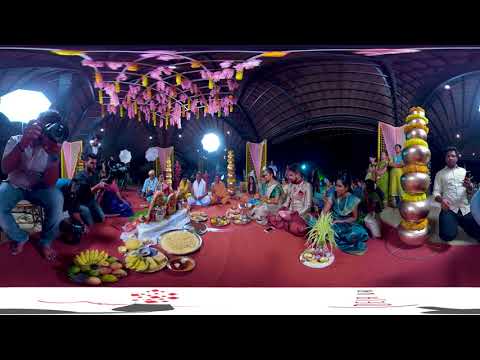The image showcases a vibrant and colorful indoor scene that depicts a ceremonial event, likely an Indian wedding or a religious celebration, given the ornate attire and decorations. The scene is framed with thick black borders at the top and bottom, intensifying the richness of the colors within. The setting features a cherry-popsicle-pink carpet or blanket sprawled across the floor, with pale blue cloths laid over it.

In the center background stands a young couple, possibly the bride and groom, with the woman in a beautiful gown and the man kneeling beside her, both facing the camera. Surrounding them are several guests, dressed in an array of vivid colors—teal dresses, light tops, white shirts, and orange garments. A notable figure to the center right is a man in a white shirt and black pants, kneeling and seemingly holding a camera.

The foreground to the left features a striking figure, a young man with a camera, seated on a high stool. His presence is marked by a bright light behind him, possibly a window. Above him hangs a floral arrangement of pink, yellow, and pale purple blossoms, adding to the exotic ambiance of the setting. This indoor space, adorned with arched windows and walls, also includes multicolored scarves hung on yellow frames in the background, enhancing the festive atmosphere.

Scattered across the floor, interspersed among the guests, are trays and plates filled with colorful food, suggesting a communal meal. Three decorative towers, reminiscent of Hawaiian leis but distinctly ornate, are visible—one prominently in the foreground and two in the center background.

Overall, the scene is a burst of psychedelic colors and joyful expressions, capturing the essence of a significant cultural celebration in a visually striking manner.